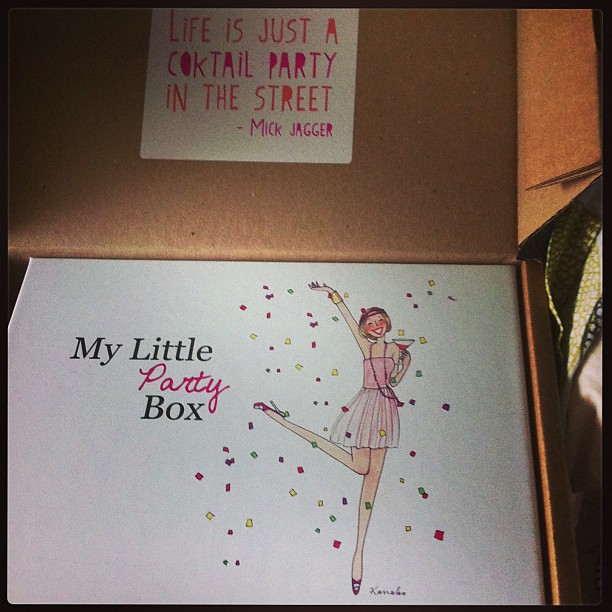The photograph shows an open brown cardboard box with a white sticker in the middle of the lid that reads, "Life is just a cocktail party in the street" - Mick Jagger. Inside the box is a white box labeled "My Little Party Box." The white box features a cheerful illustration of a woman in a pink dress, adorned with a beaded necklace, and red cheeks. She is holding a martini glass, with one leg kicked up and an arm raised in celebration, surrounded by colorful confetti. She also sports pink high heels. The overall image conveys a festive and joyous atmosphere, highlighting the theme of a lively party.